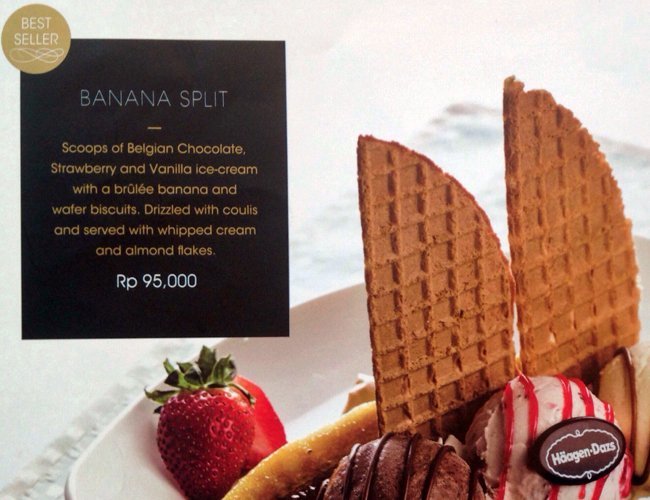The promotional image showcases a delectable Haagen-Dazs banana split dessert elegantly arranged on a white porcelain square plate, set atop a white placemat on a white table. The dessert features a single, vibrant red strawberry with green leaves, positioned prominently on the plate. To the right of the strawberry, there are three perfectly scooped ice creams: Belgian chocolate, strawberry, and vanilla, each drizzled with flavorful syrup. Two waffle cookies are artfully standing upright in the ice cream, adding a crunchy texture to the creamy treat. The lower right corner of the plate features a small brown oval logo with the name Haagen-Dazs, denoting authenticity and quality.

In the upper left corner of the image, there's a gold circle with white text that reads "Best Seller," drawing attention to the dessert's popularity. Below this, within a black rectangle, is the dessert’s description in stylish text. The blue print headline says "Banana Split," followed by a detailed description in gold print that reads: "Scoops of Belgian Chocolate, Strawberry, and Vanilla Ice Cream with a Brûlée Banana and Wafer Biscuits drizzled with coulis and served with whipped cream and almond flakes." The description is completed with white text stating "RP 95,000," perhaps indicating the price. The image is crisply composed, balancing the text elements with the mouth-watering visual of the dessert, making it an enticing advertisement for Haagen-Dazs’s best-selling banana split.